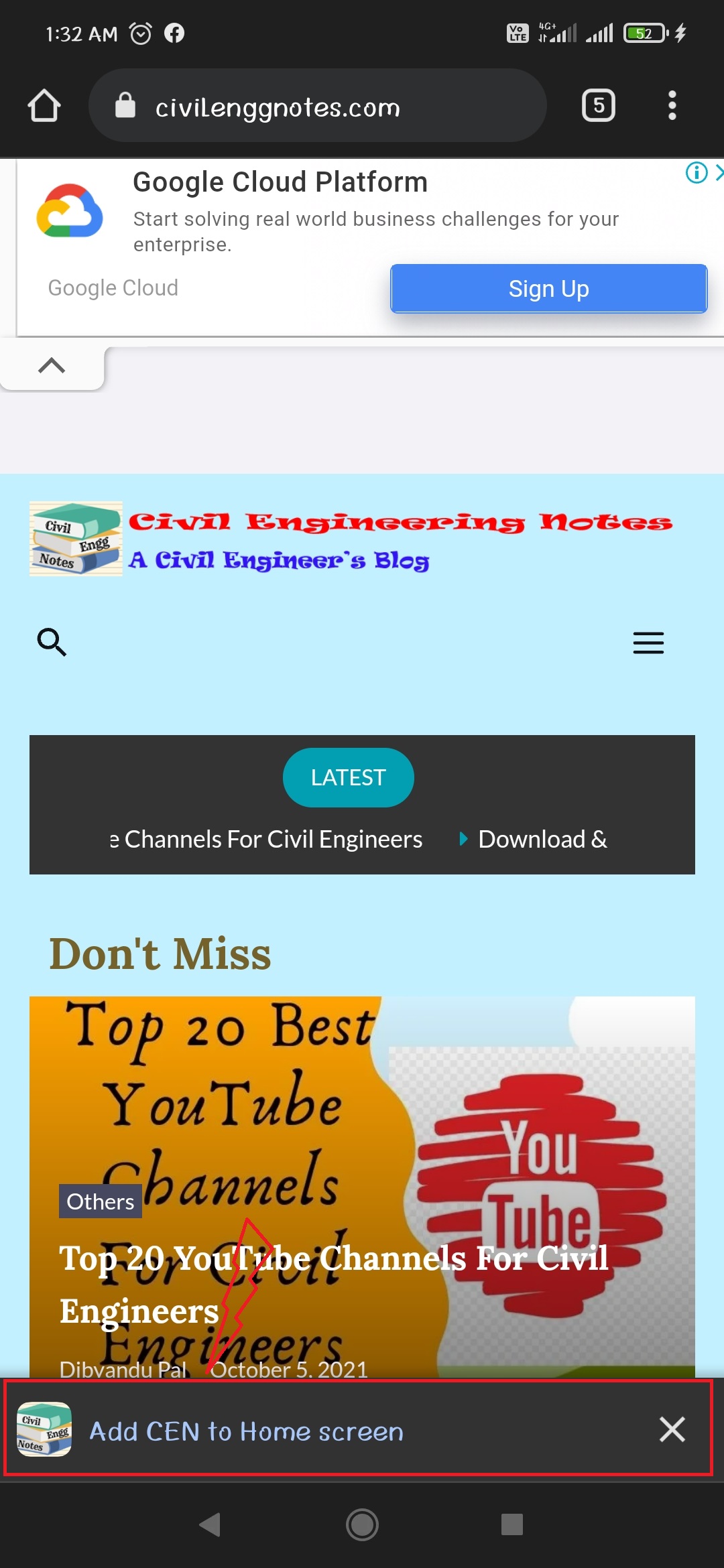At 1:32 a.m., a user is seen browsing civilenggnotes.com on their smartphone, evidenced by an alarm clock icon and a 52% battery indicator at the top of the screen. The phone is connected via LTE and features a home button. The URL bar shows a secure connection (indicated by a lock icon) and mentions five open tabs.

Below the URL bar is an advertisement for Google Cloud Platform, including a cloud logo and a promotional message encouraging users to "start solving real-world business challenges for your enterprise" with a blue 'Sign Up' button.

The website's design is characterized by a powder blue background, featuring three stacks of books with a garish red font resembling cartoon styling. The site title reads "Civil Engineering Notes" in a problematic layout, with a subtitle in blue proclaiming, "A Civil Engineer's Blog." A search field and hamburger menu are located below this title. 

A black field displays a capsule-shaped button labeled "Latest," surrounded by channel options and a partially cut-off "Download" button. Below this is an olive-colored text section stating "Don't Miss," followed by a mustard brown field with a wavy line on the left, proclaiming "Top 20 Best YouTube Channels for Civil Engineers." Adjacent to it, a YouTube logo is backed by a red scribbled circle and a gray and white checkered pattern.

Overlaid on this is white text on both sides announcing "Top 20 YouTube Channels for Civil Engineers." Additionally, a red lightning bolt directs attention toward a red rectangle highlighting the stacked books image near the bottom, promoting an option to "Add CEN to Home Screen." The interface concludes with standard navigation buttons at the bottom of the phone.